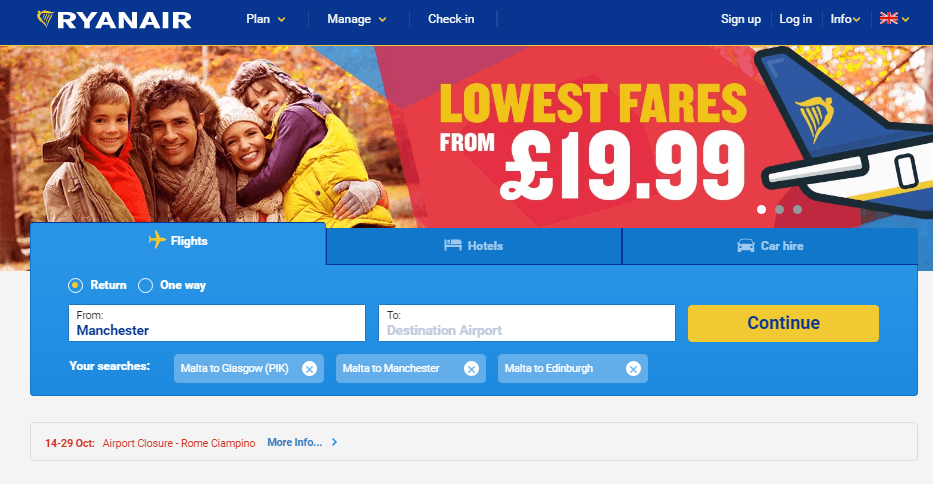This image depicts a Ryanair airline website. The top left corner features the Ryanair logo. Adjacent to the logo, a blue navigation bar spans across the top, containing several menu options. From left to right, the options include "Plan," "Manage," and "Check-In," each accompanied by a yellow arrow pointing downward. Further to the right, there are options for "Sign Up," "Log In," "Info," and a UK flag, also each with a yellow arrow pointing downward. All text in the navigation bar is written in white.

Beneath the navigation bar, there is a prominent image showcasing a family of four standing outdoors in what seems to be an autumn setting. Centered in this image is an announcement reading "Lowest Fares from £19.99." The text is stylistically varied, with "Lowest" in yellow, and "Fares from £19.99" in white and blue.

Below the image are three tabs: "Flights," "Hotels," and "Car Hire." The "Flights" tab is currently selected. To the left, a return journey option is highlighted, demonstrating a search from Manchester to a destination airport. A yellow "Continue" button is positioned at the bottom right of this section.